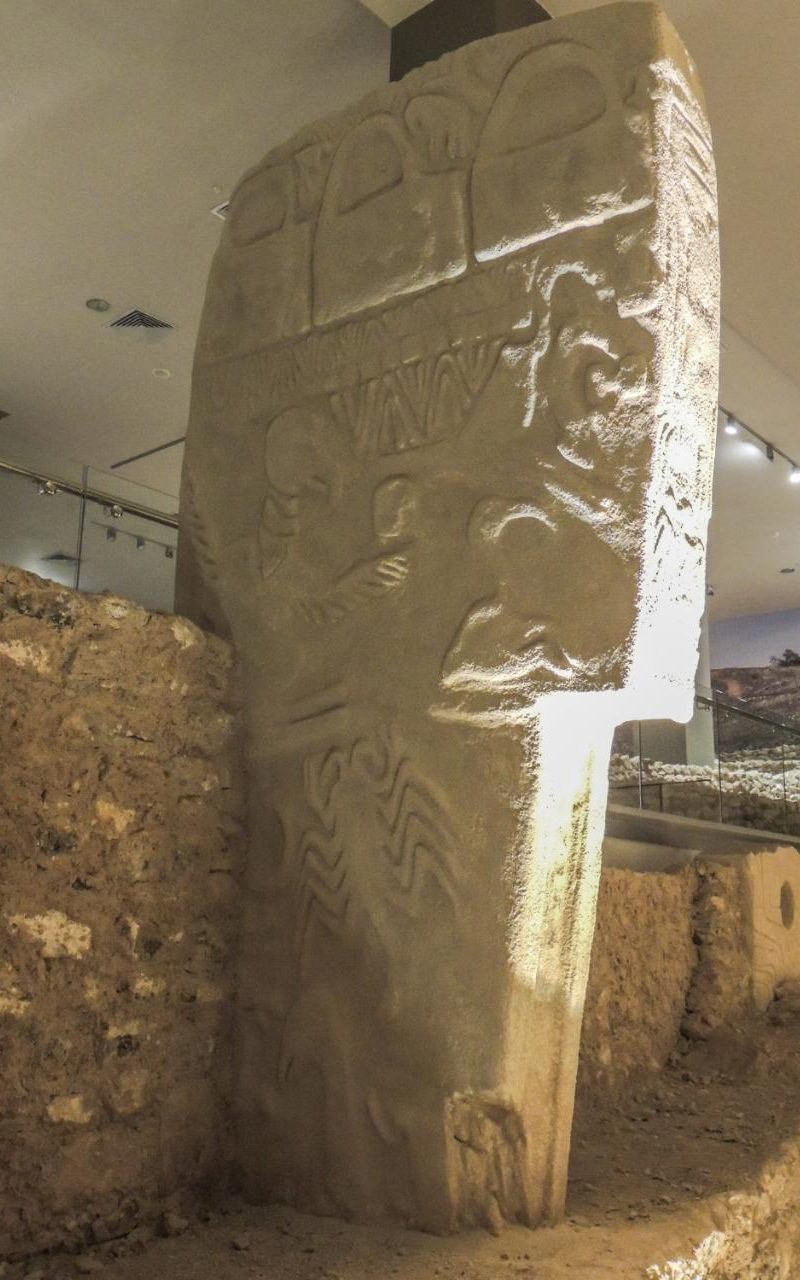This photograph depicts a tall, ancient-like vertical stone column with intricate carvings, possibly hieroglyphics in the style of Egyptian relief. The column's structure comprises a narrower bottom 40% and a wider top 60%, creating a right-angle junction between the two segments. The column is significantly thinner from front to back compared to its side-to-side width. Detailed imagery on the column includes indistinct figures, such as bird-like shapes resembling ostriches and herons, as well as a scorpion-like figure and a zigzag design.

The column is situated indoors, likely within a museum or archaeological exhibit, featuring high white ceilings and white walls. Attached to the column’s left side at around half its height is a rough stone wall. The setting includes additional granite pillars on either side and a concrete or granite floor with glass guardrails in the background, enhancing the exhibition atmosphere. White lights string across the ceiling, illuminating the entire area. The column itself is a light brown to beige color, blending with the overall clean, well-lit environment of the space, which gives off an impression of a carefully preserved and displayed archaeological find.